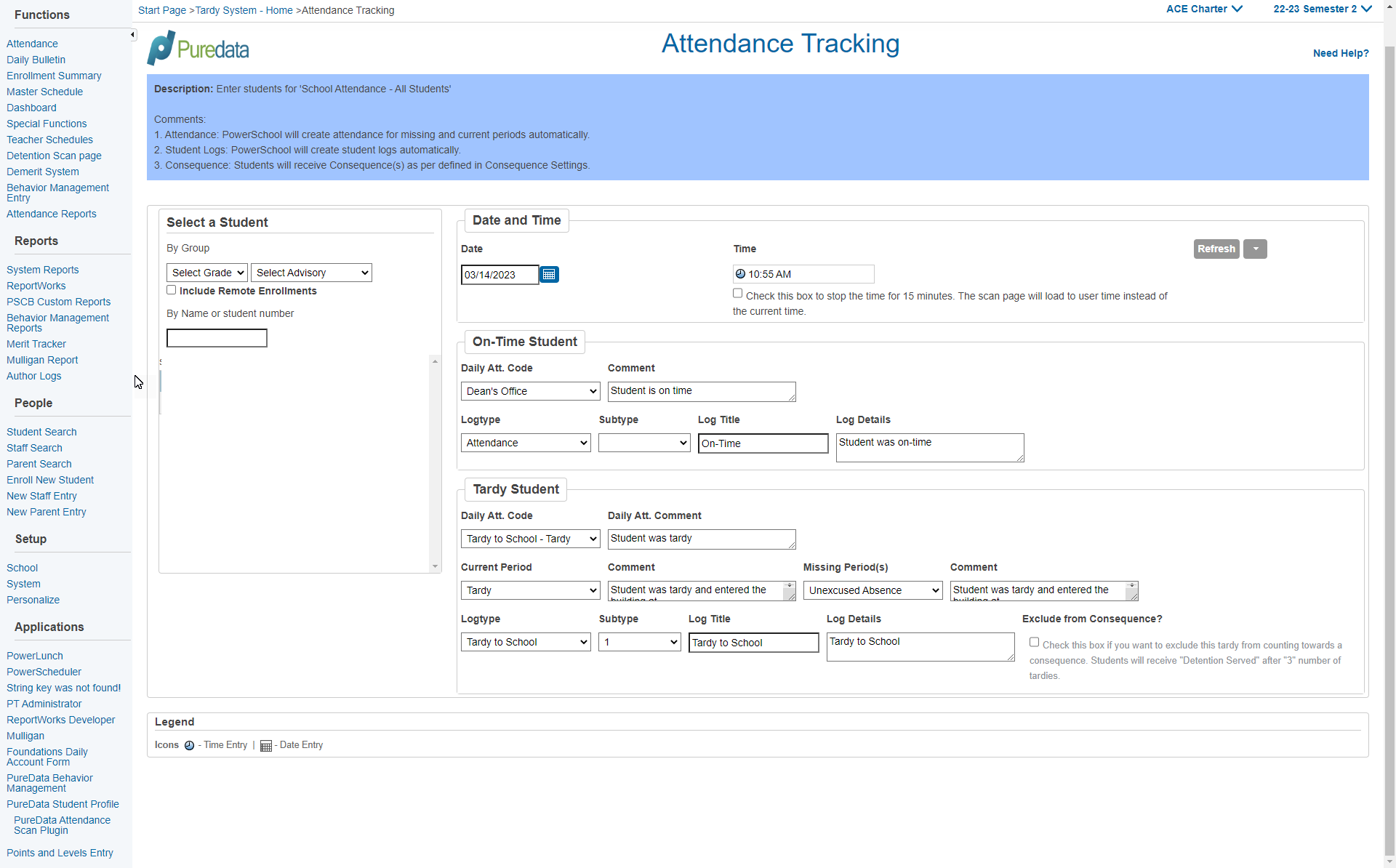Screenshot of a computer screen displaying a comprehensive school management website. The interface primarily consists of various menus, data input fields, and a detailed attendance tracking system.

### Menu Navigation (Left Sidebar)
- **Heading: Functions** (Black text, separated by a gray line)
    - **Blue text items:** Attendance, Daily Bulletin, Enrollment Summary, Master Schedule, Dashboard, Special Functions, Teacher Schedules, Detention Scan Page, Demerit System, Behavior Management Entry, Attendance Reports.
- **Heading: Reports** (Black text, separated by a gray line)
    - **Blue text items:** System Reports, Report Works, PSCB Custom Reports, Behavior Management Reports, Merit Tracker, Mulligan Report, Awesome Ops.
- **Heading: People** (Black text, separated by a gray line)
    - **Blue text items:** Student Search, Staff Search, Parent Search, Enroll New Student, New Staff Entry, New Parent Entry.
- **Heading: Setup** (Black text, separated by a gray line)
    - **Blue text items:** School System, Personalized.
- **Heading: Applications** (Black text, separated by a gray line)
    - **Blue text items:** Power Lunch, Power Schedule, String Key Was Not Found, PT Administrator, Report Works Developer, Mulligan, Foundation's Daily Account Form, Pure Data Behavior Management, Pure Data Student Profile, Pure Data Attendance Scan Plugin, Points and Levels Entry.

### Central Section (Top)
- **Top Text Items:** Start Page, Tardy System, Home, Attendance Tracking
- **Top Right Corner:** ACE Charter, Down Arrow, 22-23, Semester 2, Down Arrow
- **Horizontal Gray Line:** Extending across the section
- **Logo:** "Pure Data" symbol – the letters "P" and "D" overlap at the circle part and diverge at the tails.
- **Header:** Large blue text "Attendance Tracking" in the middle
- **Sub-header:** Small blue text "Need Help?" with a question mark on the right.

### Attendance Tracking Section
- **Header:** In a medium blue box with black bold text: "Description: Enter students for school attendance – all students."
- **Sub-items:**
    1. Attendance: PowerSchool will create attendance for missing and current periods automatically.
    2. Student Logs: PowerSchool will create student logs automatically.
    3. Consequence: Students will receive consequences as per defined in consequence settings.

### Student Selection Form
- **Left Box:**
    - Bold text "Select a student"
    - Gray line separating sections.
    - Regular text fields: By group (with drop-down arrow), Select advisory (with drop-down arrow)
    - Empty gray square with bold text: "Include remote environments"
    - Regular text: "By name or student number" and a black outline box for entering a number
- **Right Box:**
    - Long gray box for "Date and Time" with bold text at the top.
    - Below: Date "3-14-2023" and a green square with a calendar icon.
    - "Time" in bold, "10:55 AM" with a blue circle indicating time.
    - Check box to stop the timer for 15 minutes; attendance scan page will load user time instead of the current time.
    - Buttons: Gray box "Refresh" and gray square with down arrow 

### Attendance Logging Forms
- **Section: One-Time Student**
    - **Daily Attendance Code (Dean's Office) with drop-down arrow**
    - **Comment:** Student is on time.
    - **Log Type:** Attendance with a drop-down arrow.
    - **Subtype:** (Blank with a drop-down arrow)
    - **Log Title:** On time.
    - **Log Details:** Student was on time.

- **Section: Tardy Student**
    - **Daily Attendance Code:** Tardy to school-tardy with drop-down arrow.
    - **Current Period:** Tardy with drop-down arrow.
    - **Log Type:** Tardy to school with drop-down arrow.
    - **Comment:** Student was tardy.
    - **Detailed Comments:** Student was tardy and entered the building at (time).
    - **Subtype:** (1 with a drop-down arrow)
    - **Log Title:** Tardy to school.
    - **Missing Periods:** Unexcused absence with drop-down arrow.
    - **Log Details:** Tardy to school, (further details about student's entry time)
    - **Exclude from Consequence:** Check box for excluding this tardy from counting towards a consequence.

### Additional Section
- **Legend:** "Icons" including:
    - **Blue Circle with Clock Hands:** Time entry indicator.
    - **Calendar Icon:** Date entry.

The interface provides a robust set of tools for managing school attendance and student behavior, with clear sections demarcated by various text styles and colors for easy navigation.